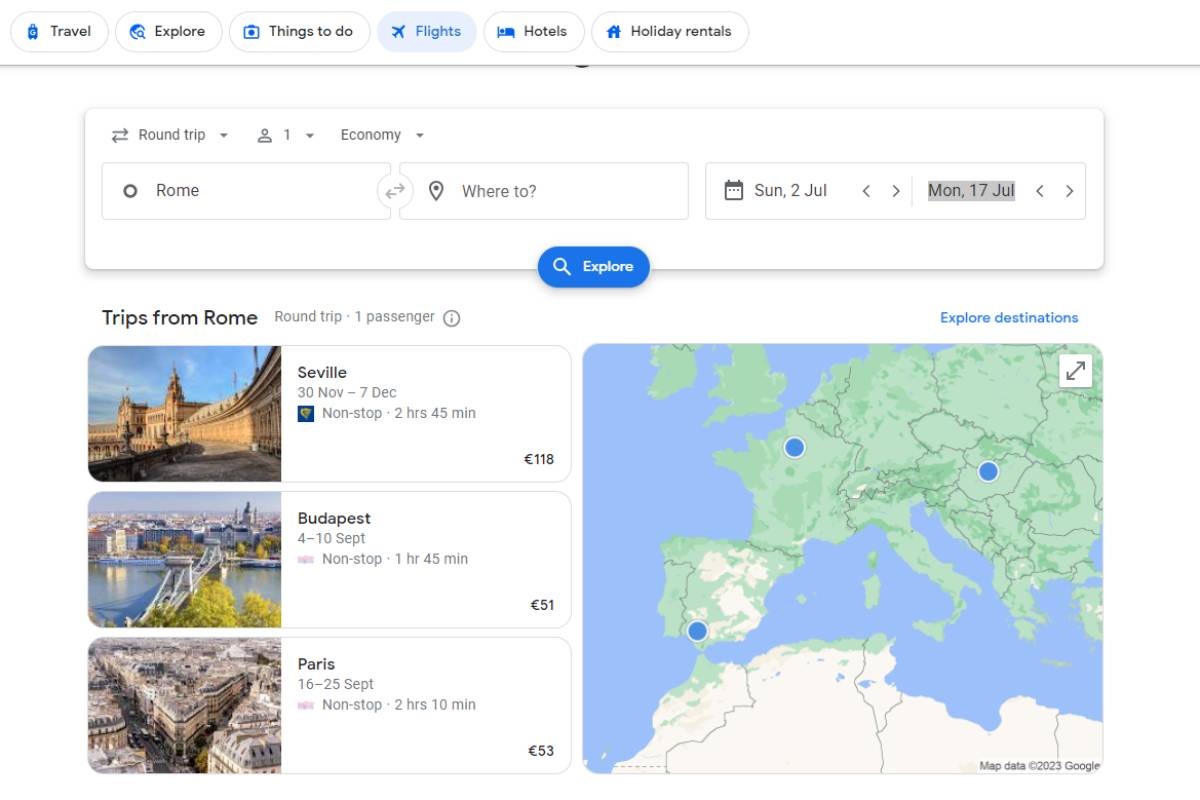The image depicts a Google Flights search page where someone is actively looking for flights departing from Rome. At the top of the page, a series of six navigational bubbles are visible. The first bubble is labeled "Travel," the second "Explore," and the third "Things to Do." The fourth bubble, which is highlighted in light blue, is labeled "Flights" and indicates the current section being viewed. Additionally, there are options to access the "Hotels" and "Holiday Rentals" sections.

The page features a clean, white layout, reminiscent of Google's interface. Prominently displayed is the flight search form, which includes options to select a "Round Trip" ticket, a passenger icon representing one traveler, and a class selection labeled "Economy." The search form specifies the departure city as Rome and provides a field for the destination. The dates selected for travel are from Sunday, July 2nd to Monday, July 17th.

Further down the page, there is a section titled “Trips from Rome,” detailing multiple potential destinations for a round trip, single passenger journey. Listed destinations include Seville, Budapest, and Paris. To the right of these listings, a map is shown marking these three cities with blue dots. The map is detailed enough to show surrounding terrains and bodies of water, including Europe and Africa. Overall, the Google Flights interface suggests that the user is planning a trip originating from Rome and is exploring various European destinations.